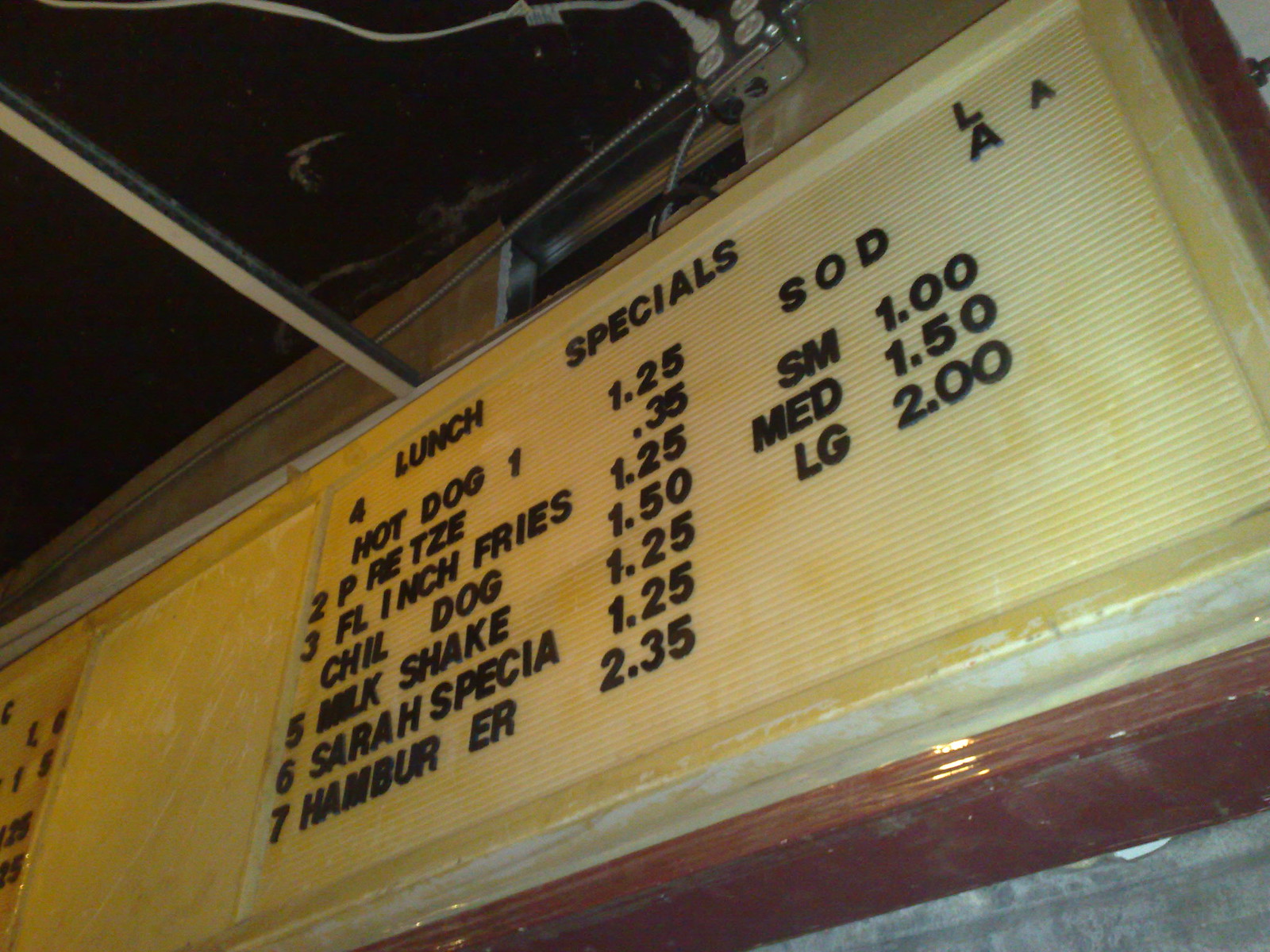In a dimly lit basement, an ancient, grime-covered sign hangs on a cinderblock wall beneath an open ceiling adorned with cobwebs and dirt. The yellow sign, framed in maroon and white, is weathered with age, its paint peeling and some letters missing. It reads "Luncheon Specials," listing nostalgic prices like a hot dog for $1.25. An image once present next to the text has faded, leaving an empty space flanked by remaining letters. Below the sign, a brand new, shiny electrical outlet contrasts starkly with its surroundings, highlighting the passage of time and the sign's decrepit state.